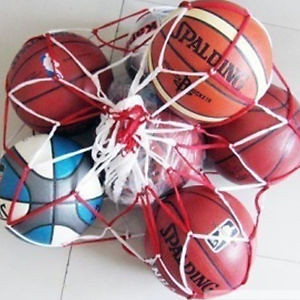The image showcases a red and white mesh net holding five basketballs, placed on a white tiled ceramic floor. Among the balls, one stands out as orange with distinctive white stripes and the Spalding logo. Another couple of basketballs are a consistent orange hue with traditional black lines, where one also bears the Spalding branding. Additionally, there's a ball noticeably different, marked by a white, blue, and gray pattern, which contrasts with the others. The variety in the basketballs' designs emphasizes their unique characteristics while the uniform mesh bag and floor setting tie the scene together.